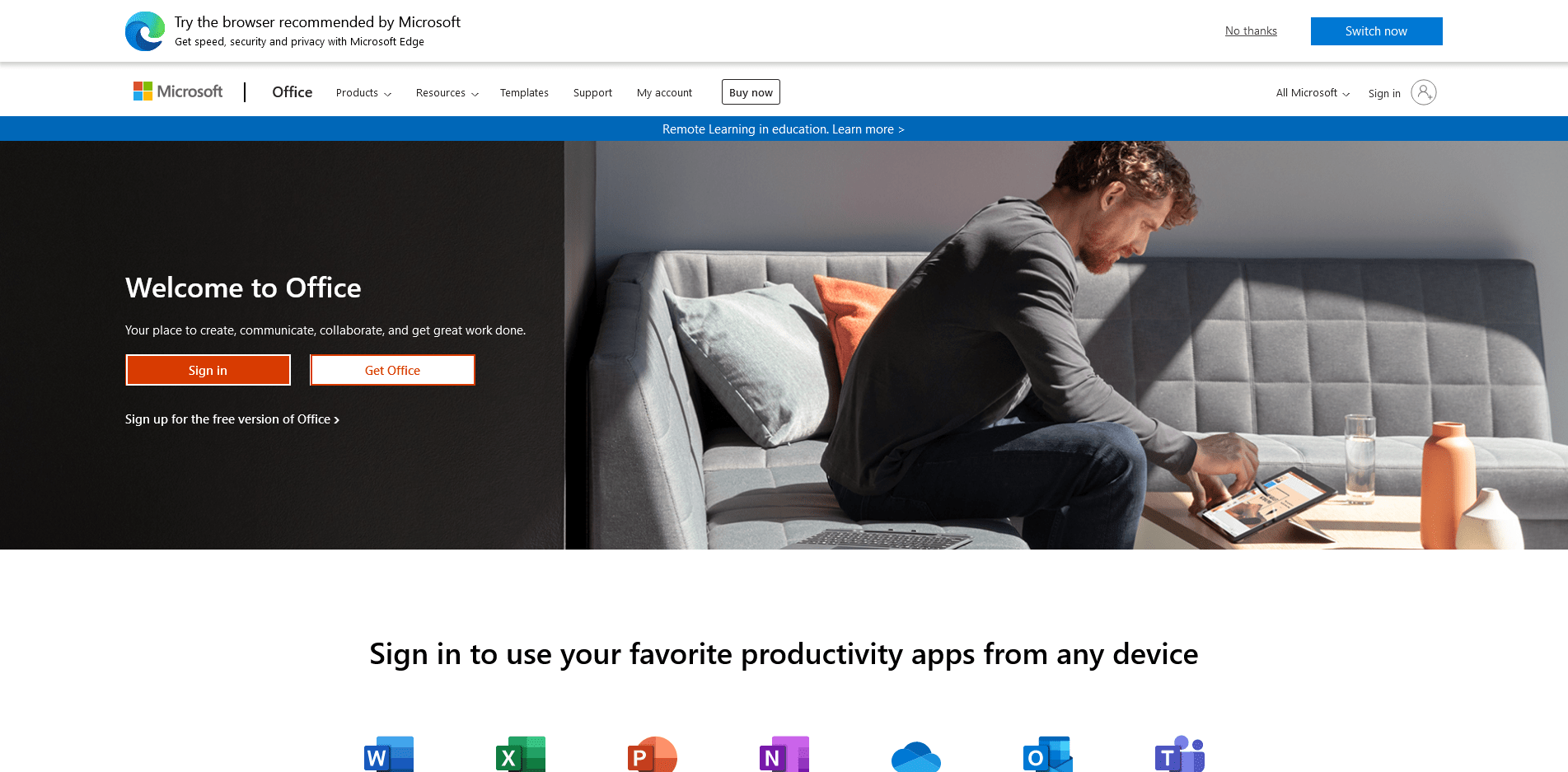This image depicts a detailed web page interface for Microsoft Office. In the upper left corner, the iconic Microsoft Edge logo is prominent, accompanied by text encouraging users to "Try the browser recommended by Microsoft," highlighting benefits like speed, security, and privacy attributed to Microsoft Edge. In the top right corner, there are two action buttons: "No thanks" and "Switch now."

Just below this section, there is a navigation bar featuring a drop-down menu labeled "All Microsoft," a "Sign in" button, and an array of links including "Office," "Products," "Resources," "Templates," "Support," and "My Account," along with a prominent "Buy now" button.

Further down, the page welcomes users with the message "Welcome to Office" and provides options to "Sign in," "Get Office," or "Sign up for the free version of Office." It also offers a link for "Remote learning in education" with a prompt to "Learn more."

On the right side of the image, there is a photo of a man using a tablet. He is seated on a sofa adorned with two throw pillows. In front of him, a table holds a glass of water and two jars, adding a casual and homey atmosphere to the setting.